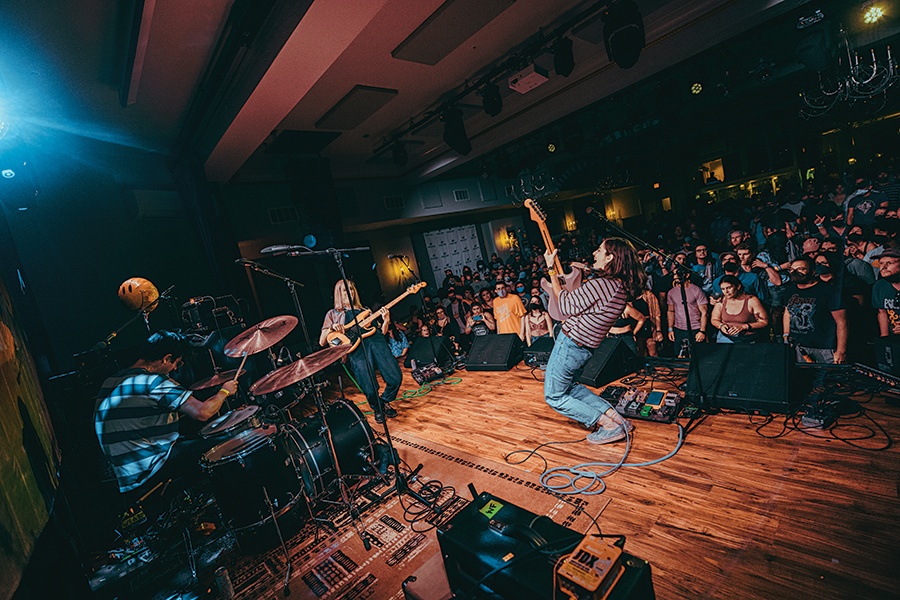This photo captures an intimate concert in a small, dimly lit room with a wooden stage and a low ceiling adorned with a chandelier. On stage, two female guitarists and a drummer create a lively atmosphere. The guitarist on the left, dressed in a black romper with a t-shirt underneath, leans backward, looking at the other guitarist in blue jeans, sneakers, and a striped maroon long-sleeve shirt who energetically lifts her guitar in the air. The drummer, positioned to the left side of the stage, plays beneath a cheerful, yellow smiley face helium balloon.

Both the stage and the performers are brightly illuminated, contrasting with the dark room filled with attentive yet subdued audience members, some wearing masks. Amplifiers, numerous cords, and speakers line the front of the stage, ensuring the music reaches the crowd standing closely together. A distinct light source from the left side highlights the scene, making the musical setup and the engaged crowd, stretching from the right to the center of the photo, clearly visible.